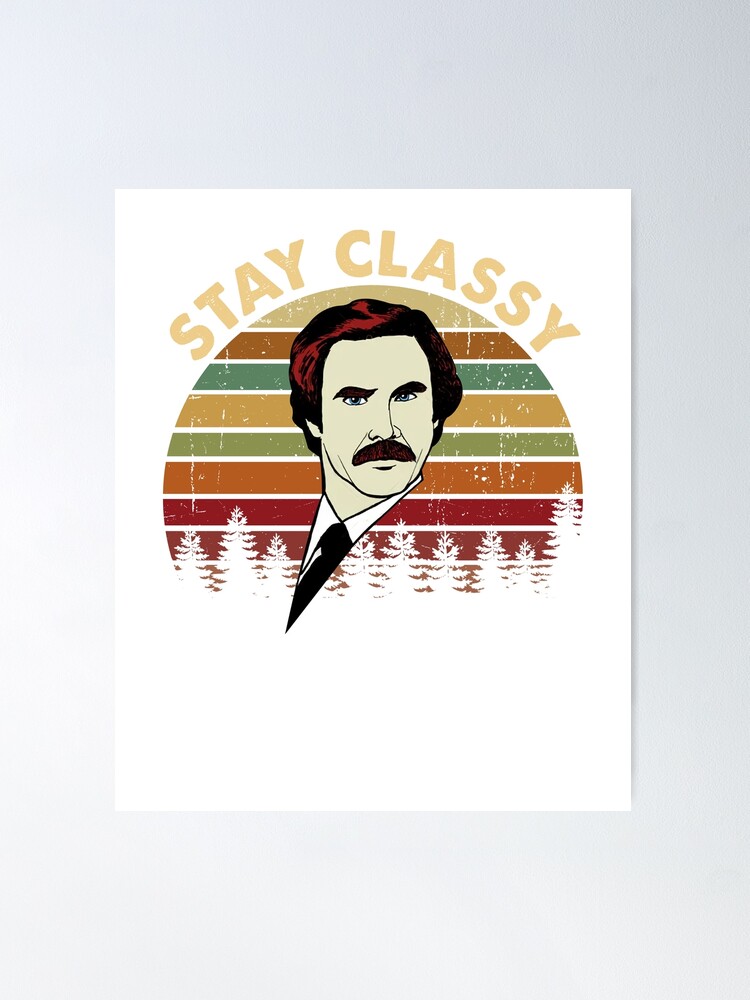This vivid drawing captures the iconic character Ron Burgundy from the movie "Anchorman." The image features a detailed, hand-drawn portrait of Ron Burgundy's face, highlighted by his signature mustache. Above the illustration, the well-known phrase "Stay Classy" is prominently displayed. Below, the drawing includes the outline of Ron's tie and collar, adding to the character's distinguished appearance. The background is adorned with horizontal lines in vibrant shades of red, orange, yellow, green, and brown, which collectively form a circular pattern around Ron's head. Further enriching the scene, pine trees are subtly depicted beneath the colorful horizontal lines, adding depth and a hint of nature to the composition.